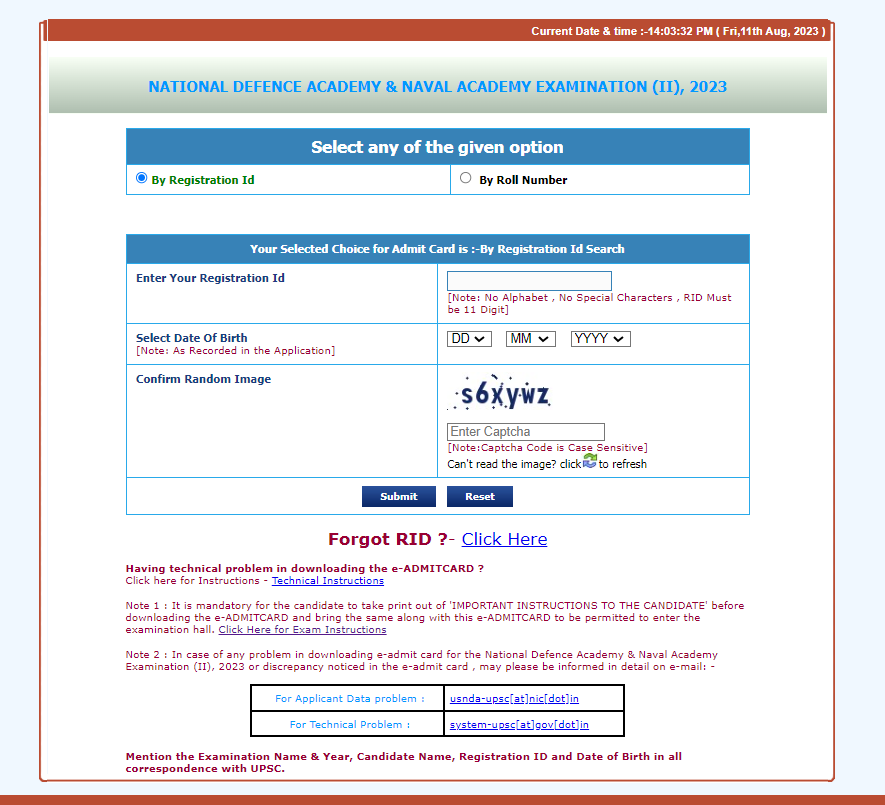The image displays an interface from a website for the National Defense Academy and Naval Academy Examination (referred to as (II) in Roman numerals), 2023. 

At the top of the page, a red bar prominently shows the current date and time: "14-03-32 PM, Friday, 11-08-2023." 

Below the red bar, there is bright blue text that reads "National Defense Academy and Naval Academy Examination (II), 2023." Notably, the word "Defense" is spelled as "Defence."

The page instructs users to select an option for downloading the admit card. The primary choice provided is "By Registration ID," which has been chosen. Below this option, another method, "By Roll Number," is mentioned.

Further down in blue text, it states, "Your selected choice for admit card is By Registration ID Search." 

The form requires users to enter their Date of Birth and to confirm a random image to proceed. On the right side of the page, there is a section dedicated to additional key information. This includes the requirement to enter a captcha and instructions for users who may have forgotten their Registration ID (RID).